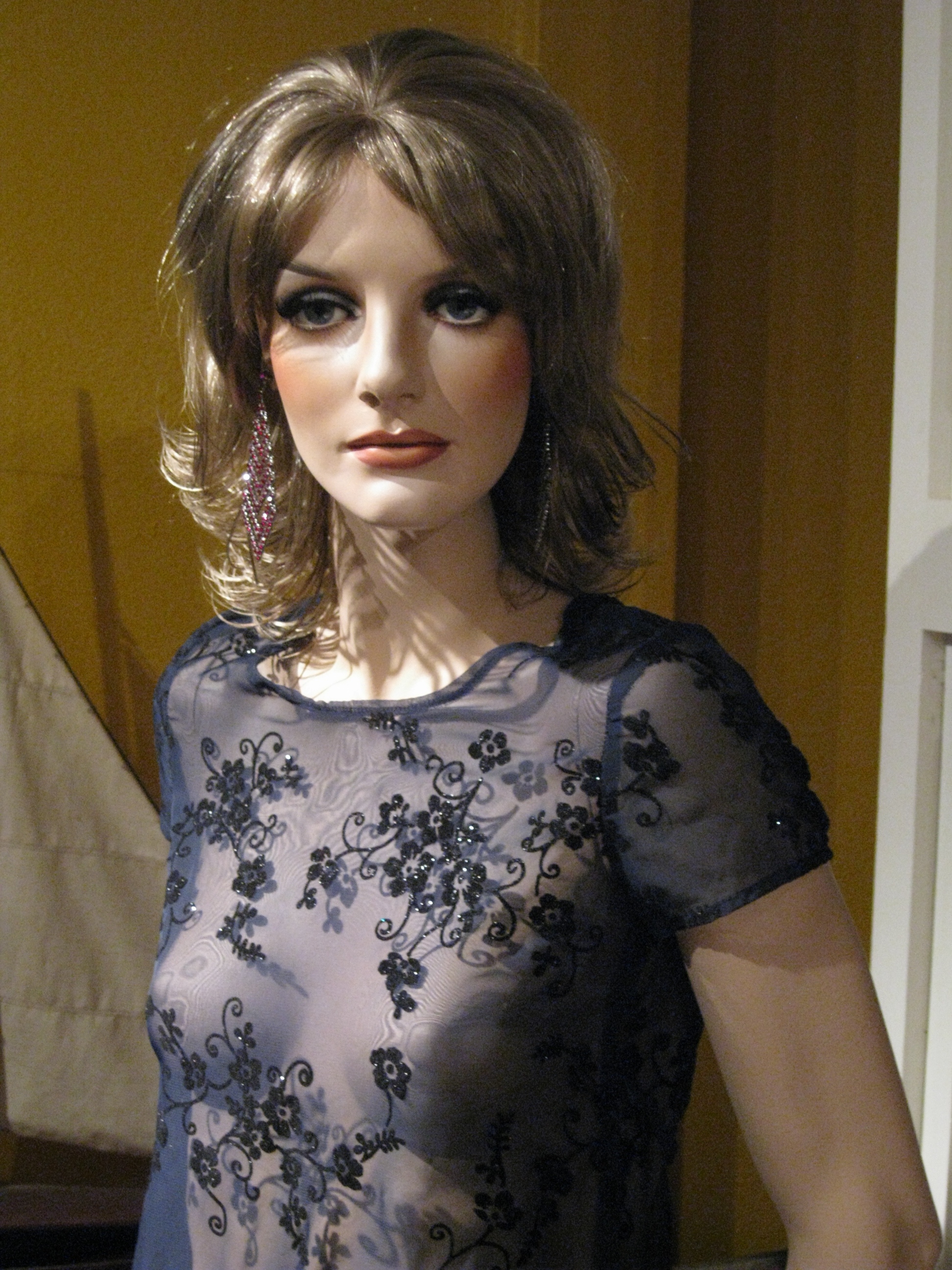The image features a highly realistic mannequin of a woman with light skin, adorned with heavy makeup including blue eyeshadow, light red lipstick, and conspicuously rosy cheeks. She sports brown, shaggy hair styled in a way reminiscent of late 60s to early 70s fashion. The mannequin is accessorized with chandelier-like purple earrings. She is dressed in a sheer, short-sleeved blue shirt with floral appliques, which allows the mannequin’s contours to be visible. The background features a yellow wall, partially obscured by the edge of a white door on the right and a white tarp in the bottom left.